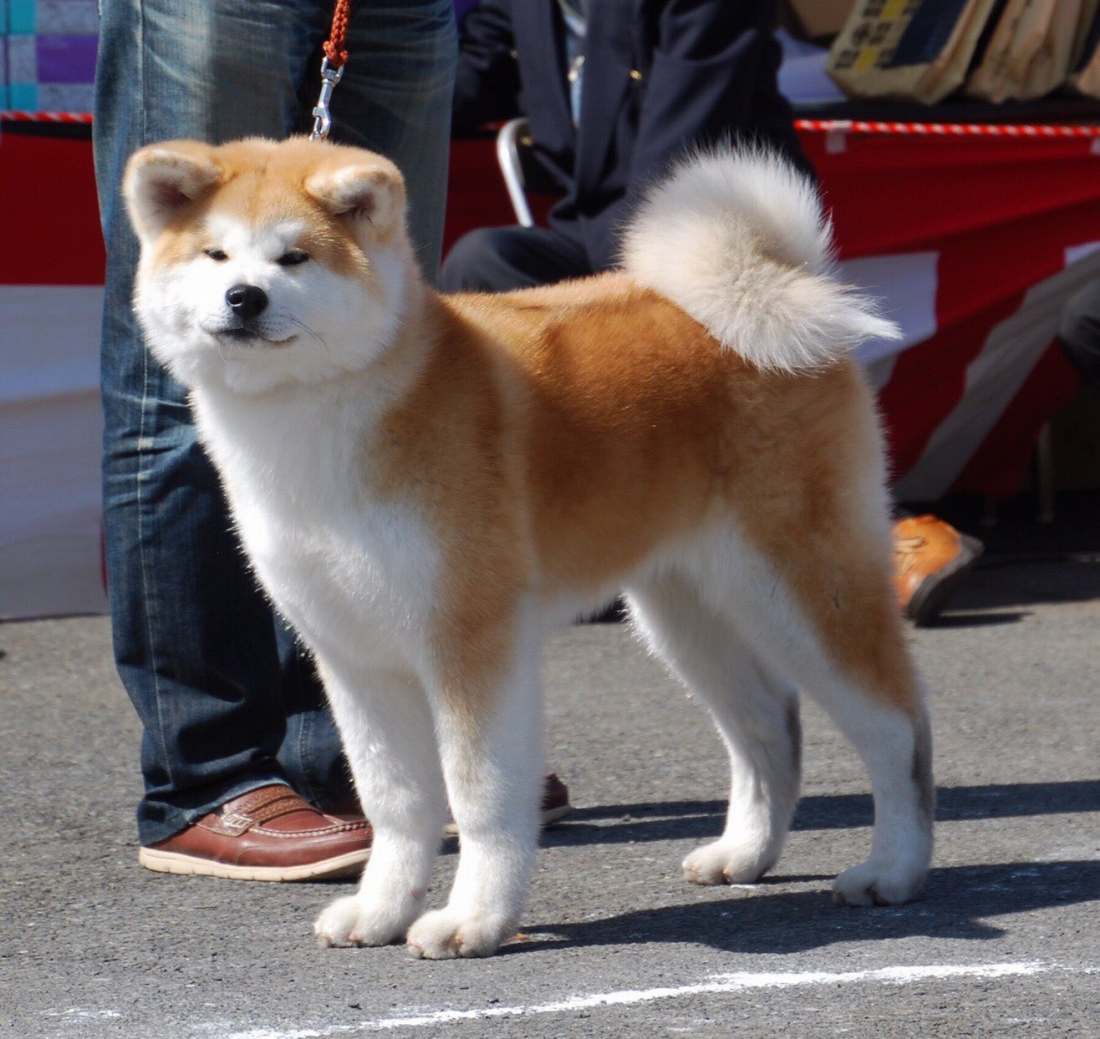The image features a light brown and white dog, possibly a Corgi, standing on a concrete pavement with a visible white line near the bottom. The dog has a golden and white coat, with a white face and a brown top of the head, neck, and back. It has a black nose and a shut mouth, gazing towards the camera. The dog's feet and chest area are white while its back and outer hind legs are a light brown. The dog is on a red leash held by its owner, whose attire includes brown loafer shoes and blue jeans. In the background, there is a red and white wall. Additionally, to the right side of the image, there is another figure's right leg in brown shoes and black pants with the foot slightly tilted. The scene appears to be set on a street with no text present. The background elements and colors such as red, white, blue, brown, black, and the leash's red are carefully highlighted, giving the impression of a dog's personal photo shoot with the handler only partially visible.